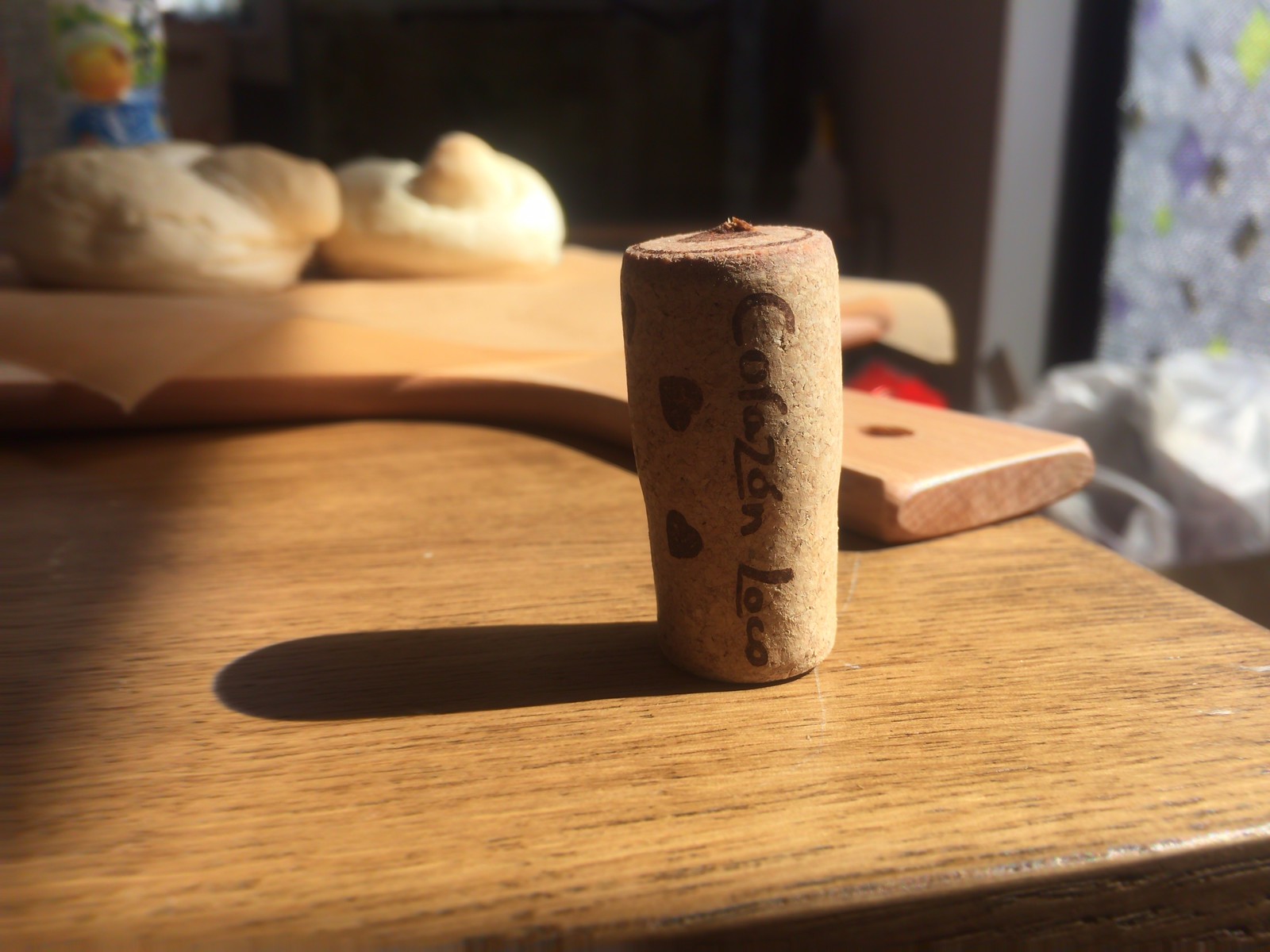The colour photograph, taken indoors, captures a wooden table seen in the landscape orientation from the edge in the foreground stretching away towards the back. A cork from a wine bottle, slightly wider at the top and narrower at the bottom, stands upright at the center foreground of the image, casting a shadow to its left due to the light coming through a window on the right. This cork includes brown horizontal and vertical text that reads "COFAZONE LOCO," alongside two black filled hearts. Behind the cork, slightly out of focus, sits a wooden pizza peel with a handle featuring a hole, likely for hanging. Resting upon the peel are two traditionally shaped challah breads with small nubs on top, their details overexposed by the sunlight streaming in, creating a white glare on their surfaces. To the right side, a flowered curtain, adorned with yellow and purple flowers and greenery, adds a touch of domestic charm, hinting at a cozy kitchen setting. The shiny, richly-grained wooden table completes the warm, homely atmosphere.